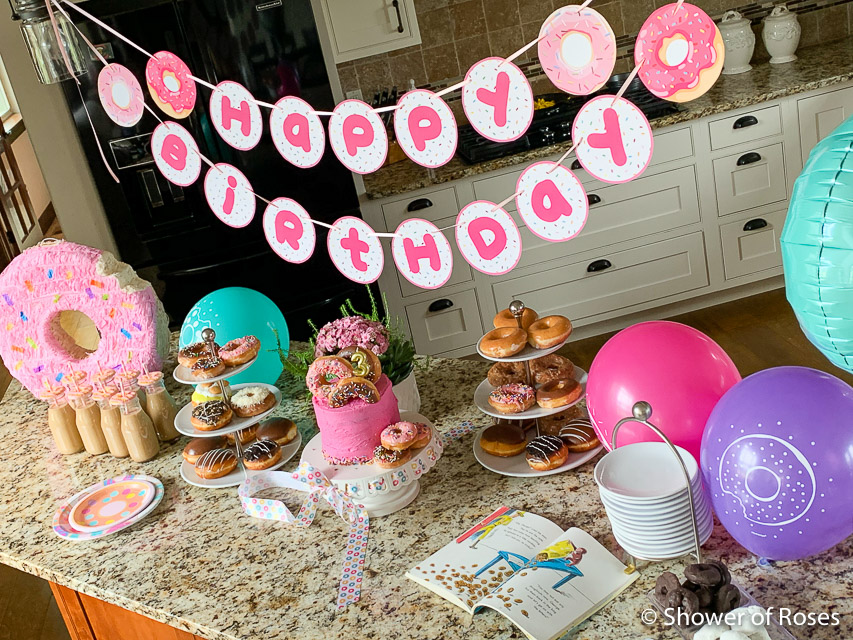The photograph captures a lively birthday party setup in a residential kitchen, centered around a joyful "Happy Birthday" banner in bubbly pink letters adorned with paper doughnut cutouts. Below the banner, the kitchen counter is festooned with a feast of treats, highlighting a pink cake adorned with the number three and three doughnuts, and two three-tiered plates brimming with doughnuts on either side. A prominent doughnut-shaped piñata and several old-fashioned milk glasses with straws, possibly filled with chocolate milk, add to the whimsical setting. The spread includes a stack of both paper and ceramic plates, pink flowers behind the cake, and an open Curious George book on the countertop, contributing to the festive atmosphere. The background showcases typical kitchen elements like cabinets and a refrigerator, adding a homey touch to this delightful celebration.